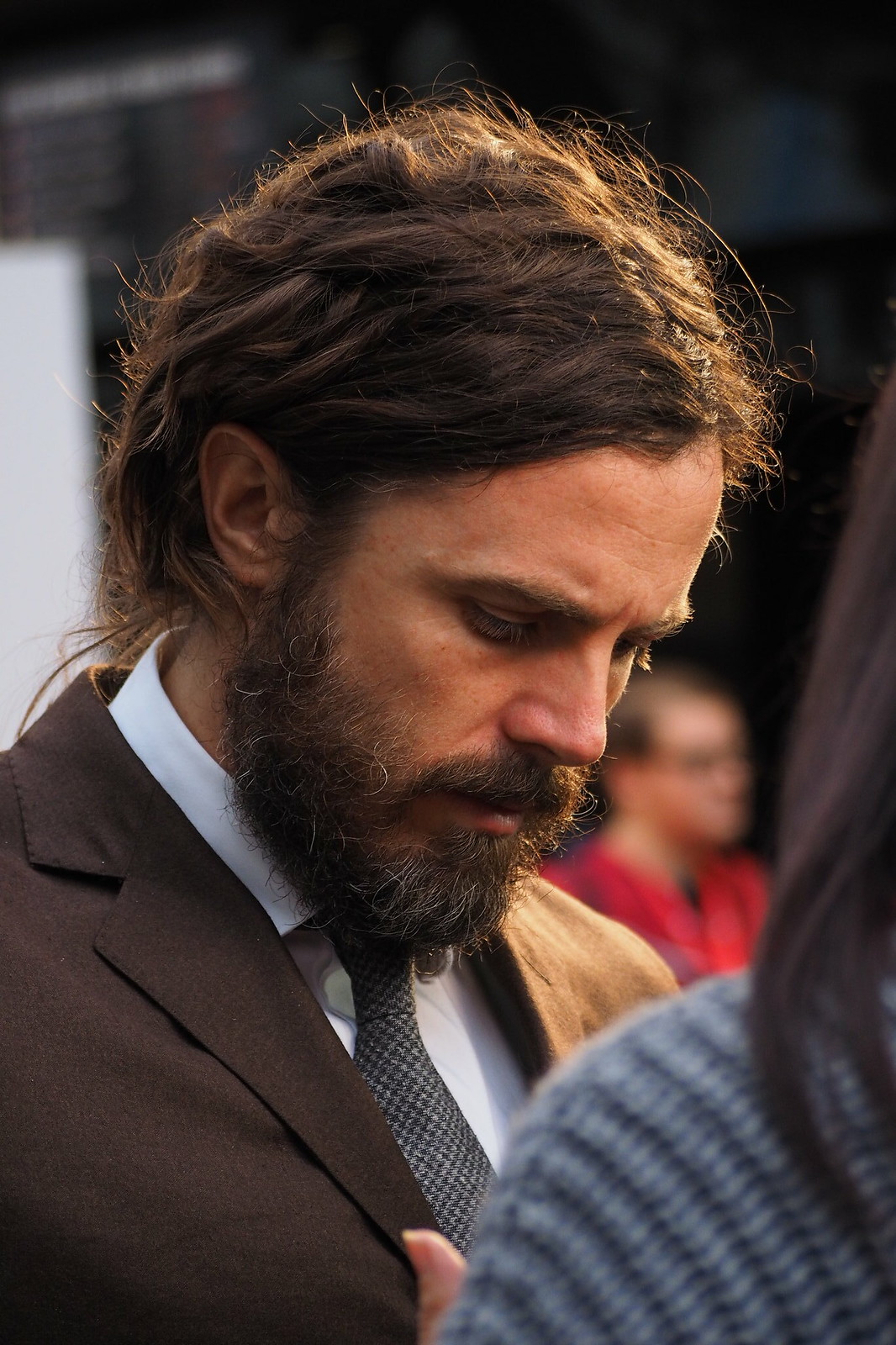The photograph features a man, likely in his late 20s to early 30s, with a solemn expression as he looks down. He has long, unkempt yet stylish hair that's pulled back into a ponytail, and he sports a scraggly, thick beard with some white strands. Dressed in a dark brown suit jacket, he pairs it with a white collared shirt and a gray, black, and white patterned tie. His attire and demeanor suggest he could be an actor, possibly even Casey Affleck, the younger brother of Ben Affleck. Surrounding him are blurred figures, including a woman in blue and a man in an orange sweater. Additionally, a man in the far corner of the image wears a red and blue striped jacket. The scene appears to be at a formal event or ceremony.